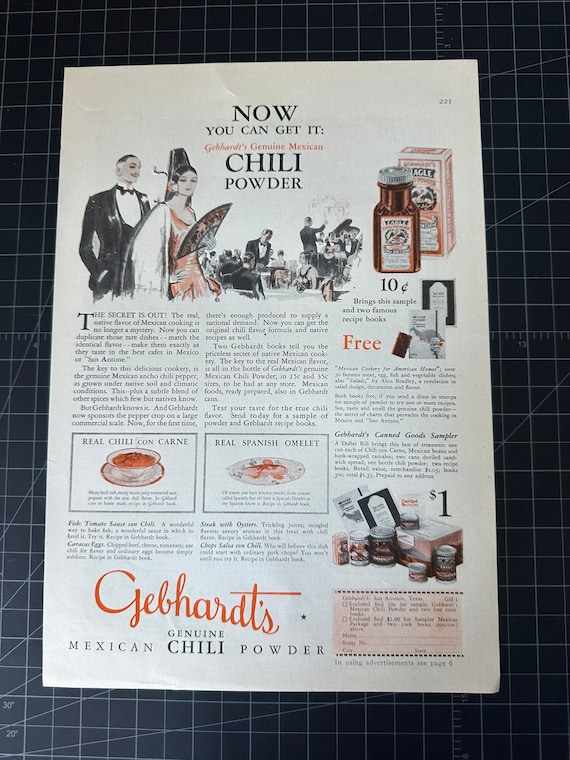This vintage advertisement from the 1940s or 1950s promotes Gebhardt's Genuine Mexican Chili Powder, capturing the elegance and charm of its era with sophisticated illustrations and detailed descriptions. Dominating the page, the ad announces in bold letters, "Now you can get it, Gebhardt's Genuine Mexican Chili Powder." A refined woman in an evening gown, holding a Japanese fan, stands prominently in the foreground, her hair elegantly pulled back. Behind her, a man in a tuxedo and bow tie, likely a waiter, emphasizes the classy, old-style restaurant setting filled with patrons. The ad showcases a photograph and drawings of the chili powder, priced at just 10 cents, and highlights various recipes such as real chili con carne and real Spanish omelet. Additionally, it mentions that the chili powder unlocks the "real native flavor of Mexican cooking." The bottom of the advertisement features further text extolling the blend of genuine Mexican ancho chili pepper with other secret spices, aimed at recreating the flavors found in the finest cafes in Mexico and San Antonio.